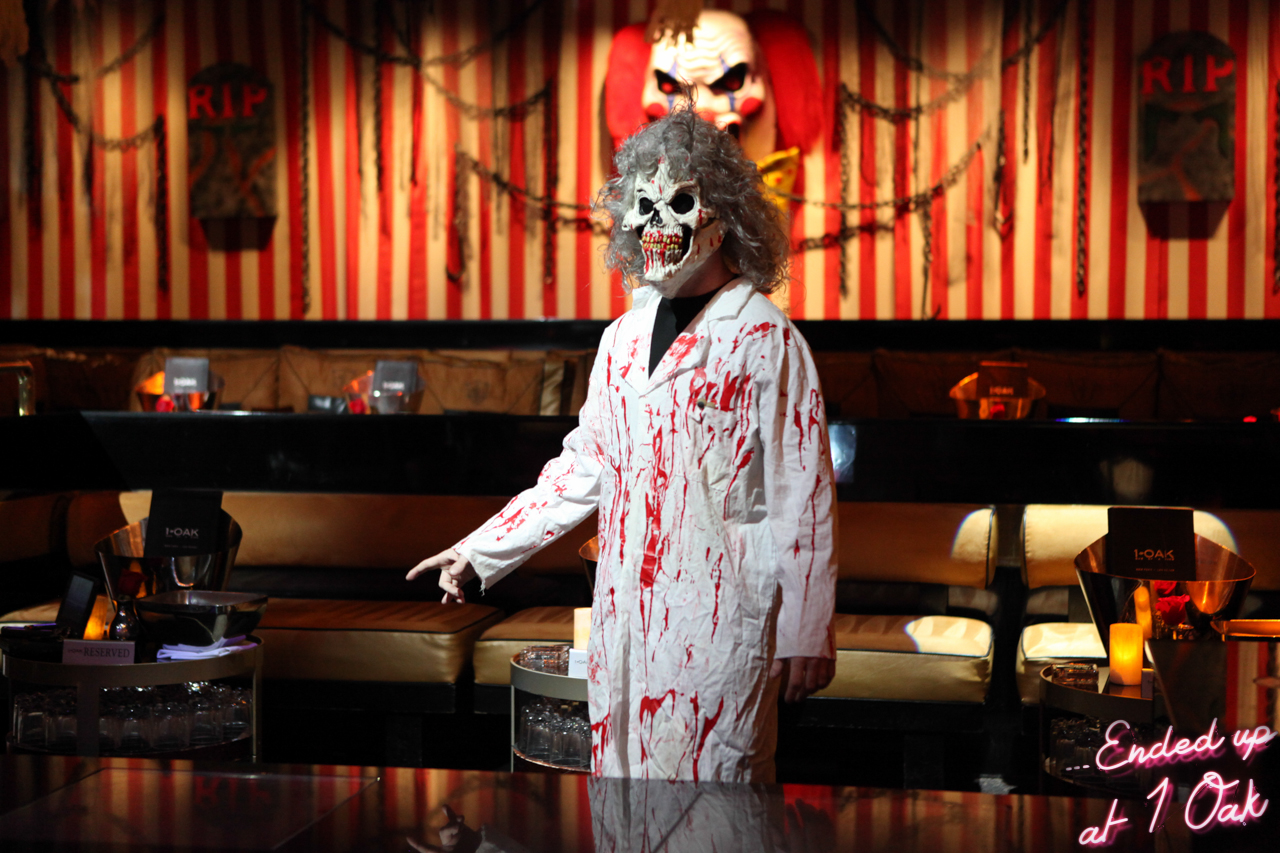A chilling image captures a person dressed as a demonic figure, standing in what appears to be a theater or club decorated with spooky decor. The individual wears a horrifying skull mask with bloody teeth, accented by a curly gray wig. They are clad in a white lab coat drenched in blood splatters, their right arm extended, pointing ominously with a finger. The background features striking red and white vertical stripes, flanked by gravestone markers inscribed with "RIP." In the center, a terrifying clown image with dark eyes and vivid red hair adds to the eerie ambiance. The scene includes rows of tan seating with round tables, each adorned with metal ice buckets, black pamphlets, and white pillar candles, enhancing the unsettling atmosphere. A caption in the bottom right reads "ended up at One Oak," hinting at the venue's name.